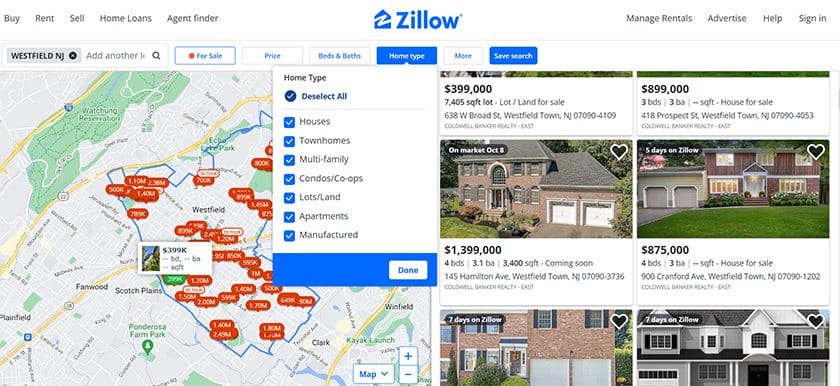On the Zillow website's desktop version, the search is filtered to show homes for sale in Westfield, New Jersey. The interface displays a map on the left, highlighting numerous listings within a compact area. On the right side, individual properties and their prices are detailed. Among the listings, there is a vacant lot listed for $400,000, encompassing 7,405 square feet. Another property, priced at $900,000, features three bedrooms and three bathrooms. A more expensive listing, priced at $1.4 million, offers four bedrooms, 3.1 bathrooms, and spans 3,400 square feet. This property is noted as "coming soon." Most visible homes appear suburban, well-maintained, and carry a high price tag reflective of the area's affluence.